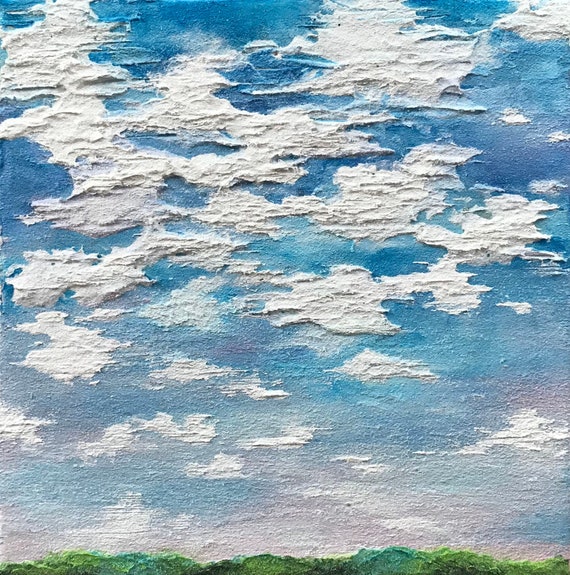In this abstract oil painting by Dick, the majority of the composition is devoted to a striking blue sky adorned with thick, textured clouds. These clouds, likely painted using titanium white, appear almost three-dimensional, as their heavily layered and sculptural nature protrudes from the canvas. The sky's deep blue shade at the top transitions into a more desaturated blue and eventually grayish hues toward the bottom, enhancing the depth and atmospheric perspective. This gradient meets a verdant landscape below, featuring various green hues depicting a forested area with curving hills. The vegetation illustrated ranges from basic green to darker tones and even mixes with blue, adding to the richness of the scene. The painting's elaborate texture, especially in the clouds, suggests the possibility of mixed media elements, making it a compelling and beautiful piece of art.